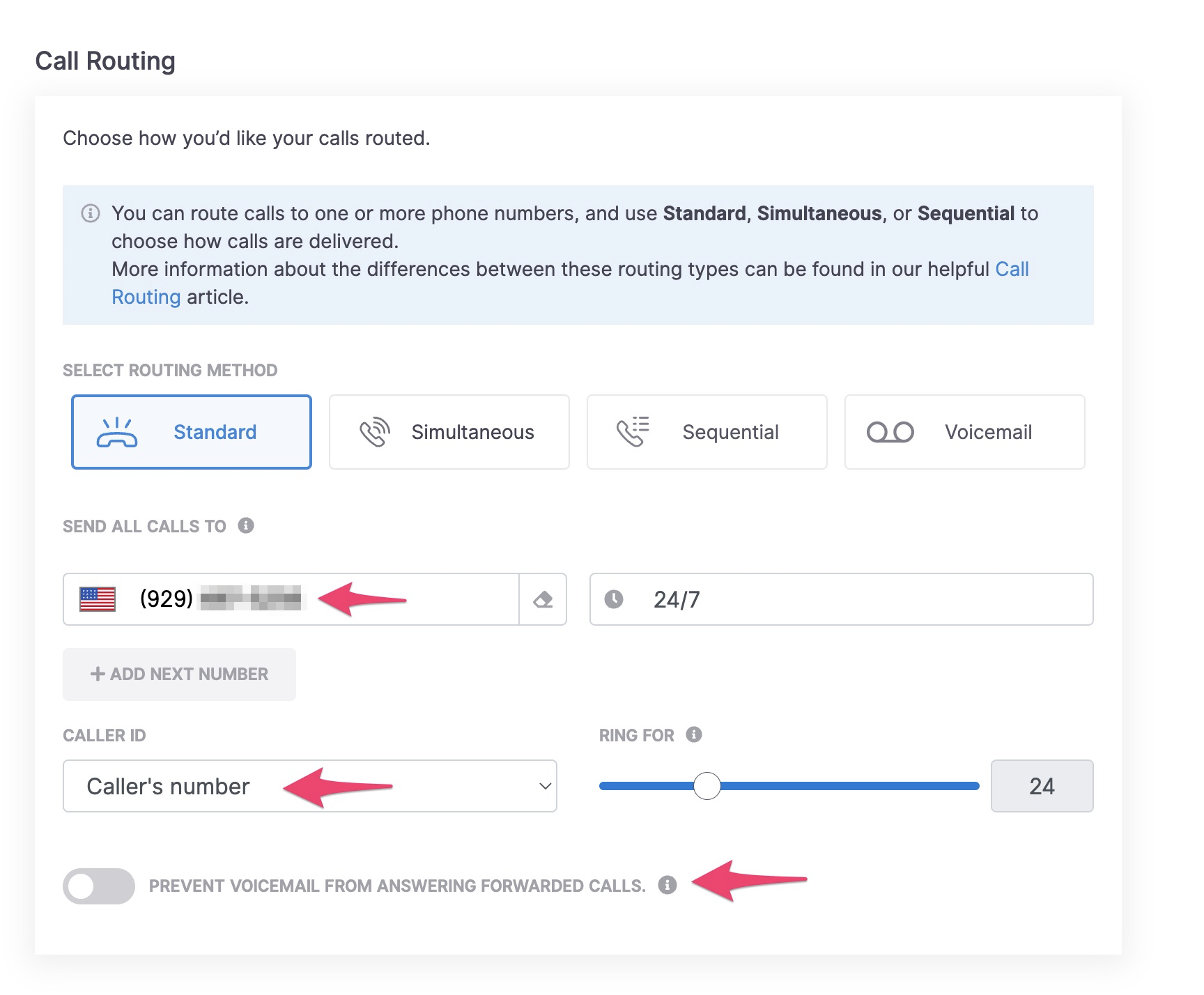The image is a detailed screenshot of a desktop interface for setting up call routing preferences, either on a website, an app, or software. At the very top, there is a heading that reads "Call Routing." Below this heading, within a white square box, there is a prompt that says, "Choose how you'd like your calls routed."

Centered within the box is a pale blue rectangular section with black text, accompanied by a small info icon. The text explains that users can route calls to one or more phone numbers, highlighting the options for call delivery methods: **Standard**, **Simultaneous**, or **Sequential** in bold text. Further, it mentions a hyperlink labeled "call routing" in blue, which presumably leads to an article providing more information about these routing types.

Under the text, users are prompted to "Select Routing Method," with visual representations of each option:
- **Standard**: Depicted by an old-style telephone handset that is currently ringing but face-down, indicating standard call routing.
- **Simultaneous**: Shown with an old-style handset leaning backward, emitting noise marks, illustrating that calls ring multiple numbers simultaneously.
- **Sequential**: Represented by an old-style phone handset alongside a list icon, signifying that calls are routed to numbers in sequence.
- **Voicemail**: Iconically, represented by the common voicemail symbol, indicating that calls can be routed directly to voicemail.

Moving further down, there are specific configurations for call routing:
1. A red arrow points towards an instruction showing a masked US phone number with the area code '929', highlighted for setting up call forwarding.
2. An option for specifying the time frame, set to "24-7."
3. A button to "Add Next Number."
4. Another red arrow points to the "Caller ID" configuration specifying "Caller's Number." 
5. The ringing duration is set to "24," which likely refers to seconds.
6. A toggle switch, currently deselected, labeled "Prevent voicemail from answering forwarded calls."

This screenshot effectively demonstrates how users can adjust various aspects of their call routing preferences within the software, offering intuitive visuals and clear instructional text to guide users through the process.